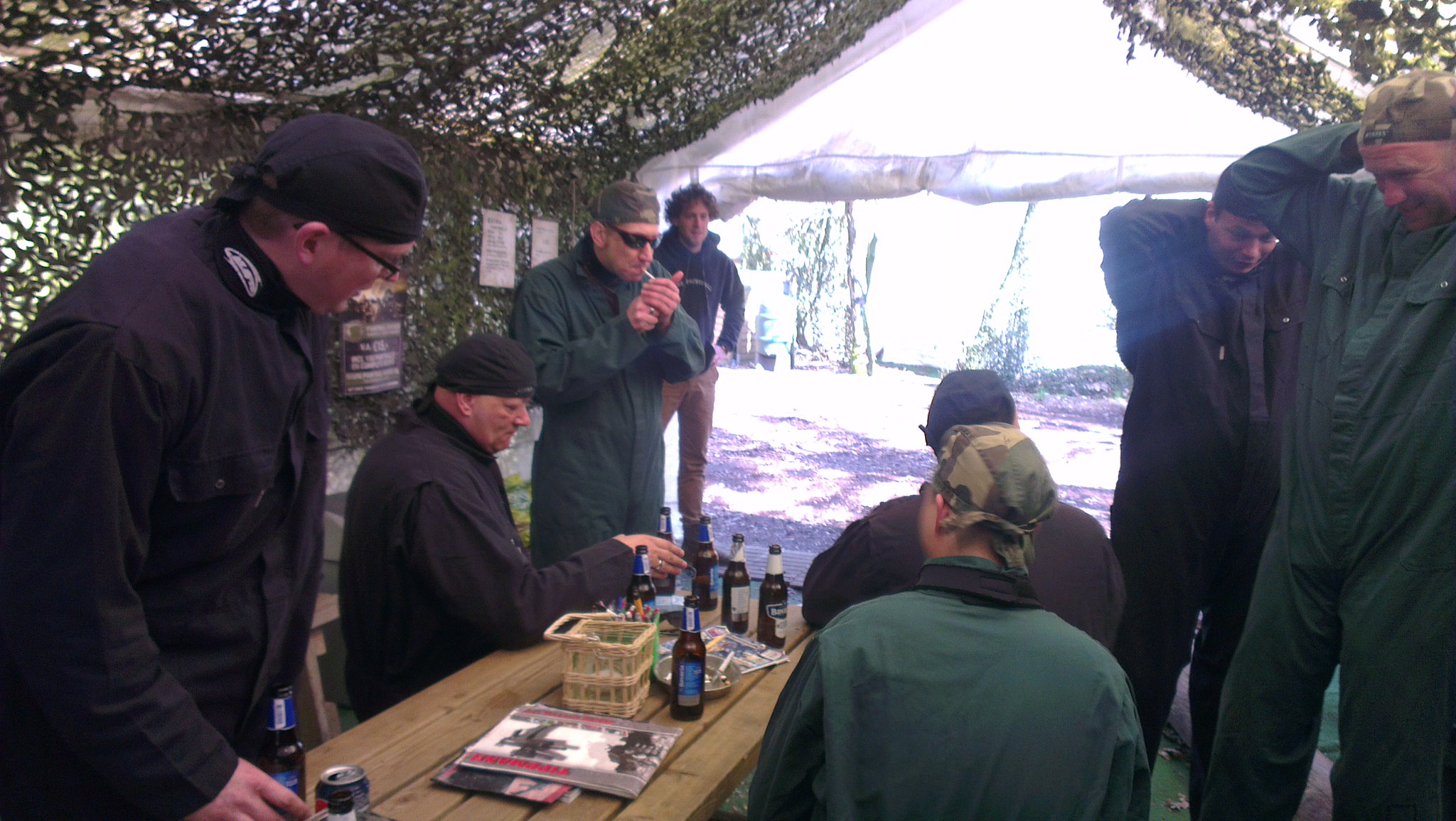The photograph captures a lively scene of eight men underneath an A-frame, camouflage-style tent constructed from brush and leaves, with sunlight streaming through a rolled-up clear drape opening in the background. The central focus is a wooden picnic table cluttered with numerous open beer bottles, an ashtray containing a lit cigarette, and scattered magazines featuring gun-related content. Also on the table is a wicker basket with a handle. On the left side of the table, three men are wearing do-rags—some black, some camouflage—while the fourth man sports a hoodie and tan pants, standing apart from the uniformed group. To the right, all four men are adorned in military-style apparel, with two facing away and two facing the camera. Their attire includes combinations of black and green jumpsuits, glasses, and distinctive head wraps. The men display a range of expressions—from laughter to relaxation. Additional details include scattered signs in various colors on the tent walls and people either sitting or standing, caught in moments of camaraderie and casual enjoyment.